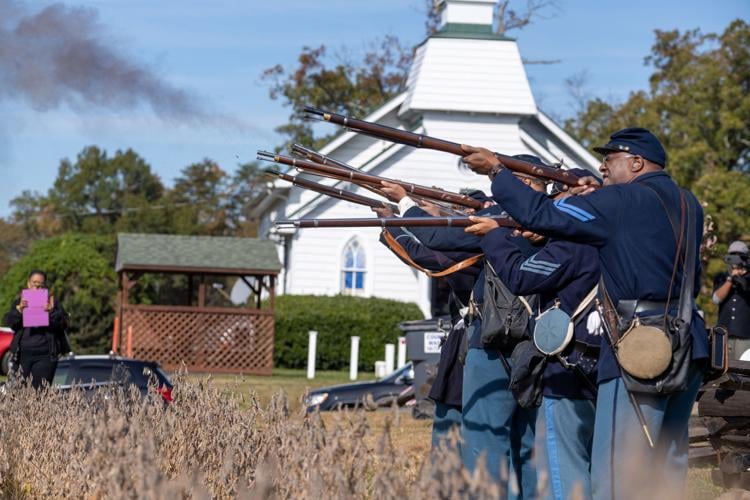In this angled photograph of a battle reenactment, a line of approximately six African American men dressed in Civil War Union uniforms is prominently featured in the foreground. Each soldier is clad in a navy blue jacket with distinctive blue stripes on the arms, paired with lighter blue pants also striped, and dark blue hats. They carry water canteens—one brown and one blue—and hold brown long muskets, from which black smoke billows as they fire into the air towards the left. Dry, brown wheat plants stretch behind them.

In the background, a traditional white southern Baptist church stands out, characterized by its white angled roof, chimney, and arched windows with white trim. Suburban trees and a lean-to structure are also visible near the church. To the left, a woman dressed in black pants and a jacket holds a purple notepad. Near the scene, various cars and a green dumpster can be seen, adding modern contrasts to the historical display.